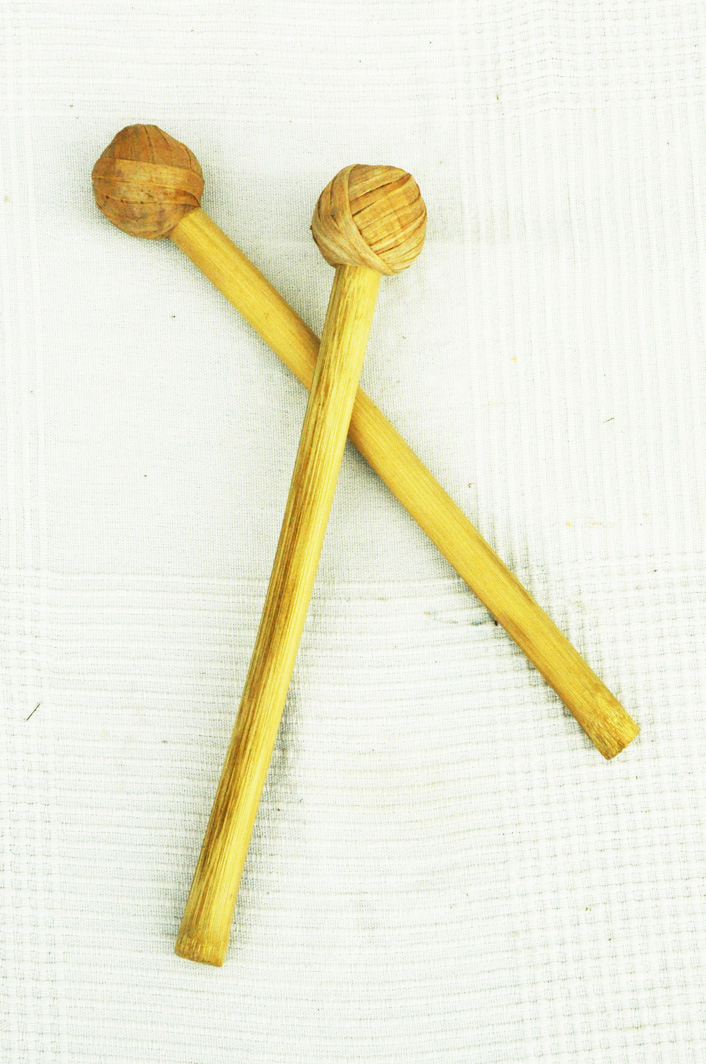The image depicts two yellowish-colored percussion mallets, potentially made of wood or bamboo, arranged on a white piece of fabric. Each mallet features a round, intricately wrapped or woven impact end, possibly covered with material or tape. The mallets are positioned with one lying horizontally and the other placed diagonally across it. The white fabric underneath them, resembling cheesecloth or a throw blanket, features a subtle pattern of small, recessed squares on the right side. The photograph, taken indoors, captures the mallets from an overhead perspective, emphasizing their craftsmanship and texture.